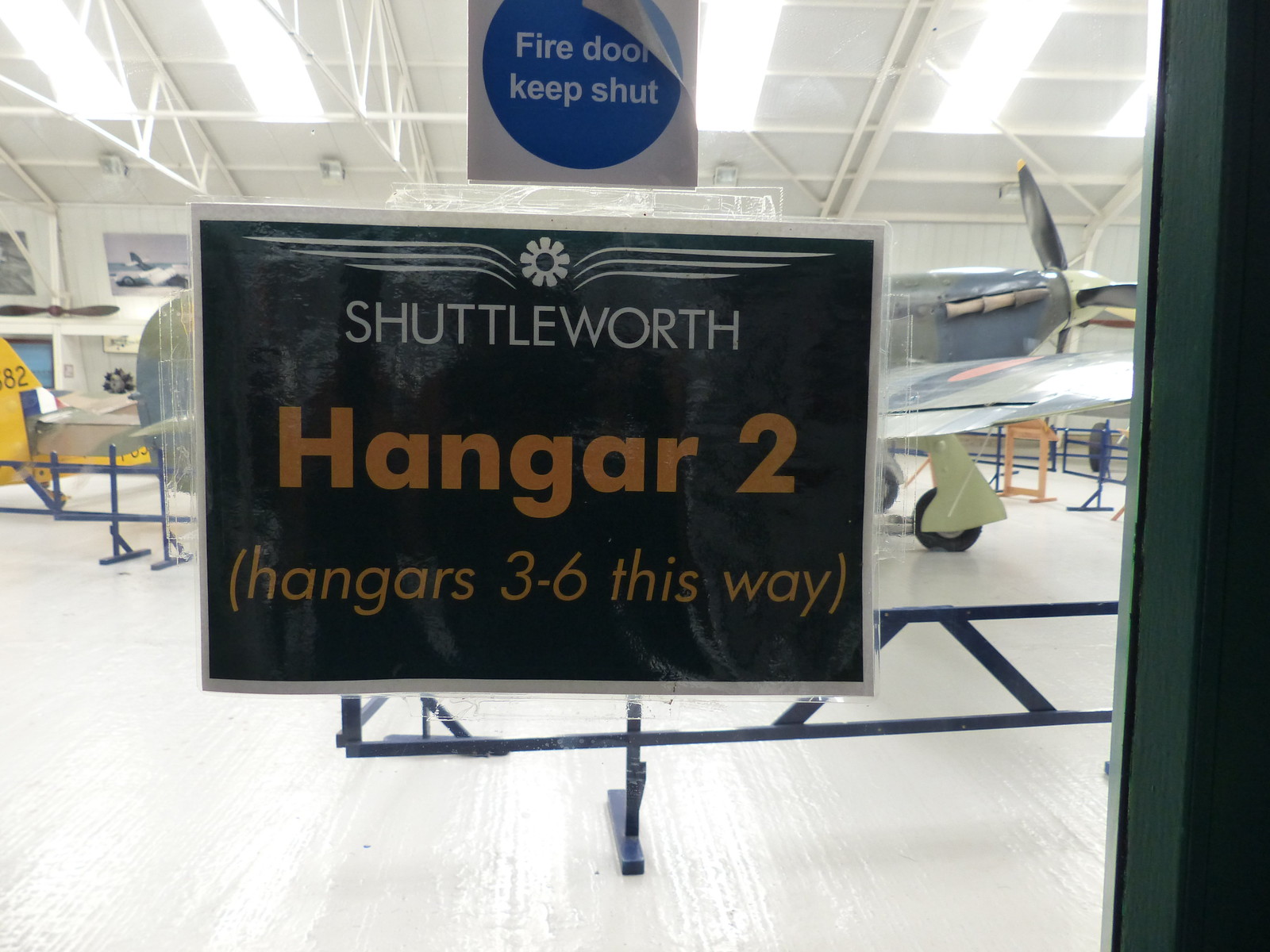The photograph captures the interior of an airplane hangar viewed through a window on a door. Dominating the center of the image is a sign affixed to the door. The top part of the sign features a blue circle on a gray background with the white text "Fire Door, Keep Shut." Below this, against a black background, is the name "Shuttleworth" in white capital letters, accompanied by a minimalist logo consisting of a center circle with single-line wings extending to the sides. Below this, "Hangar 2" is printed in bold orange letters, and beneath that, in smaller white text within parentheses, it reads "hangars 3 to 6 this way." Beyond the sign, the hangar itself displays its structural details, including lights and metal struts spanning both horizontally and vertically. Visible inside the hangar are several airplanes, including a single-engine plane prominently featuring its right wing, and another aircraft with a yellow tail fin further in the background. The scene is well-lit, possibly from skylights, and there are metal barriers around the planes, suggesting they might be part of an exhibit.